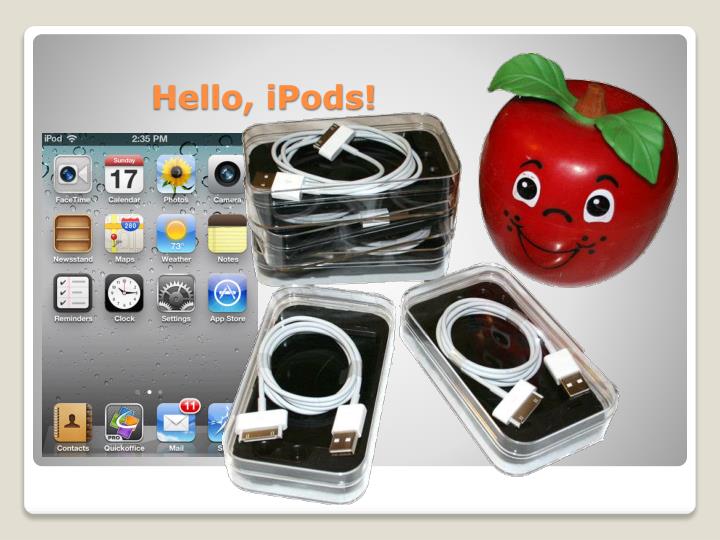This advertisement features a gray background with a headline in bold orange text that reads "Hello, iPods!" at the top. Dominating the central part of the image, there are stacked clear plastic cases containing charging cords for iPods, explicitly visible with white cables on top. To the far left of the image, there is a depiction of an iPod screen displaying a classic layout with multiple app icons arranged in rows, reminiscent of an older iPod interface. The iPod screen illustration includes a time display at the top and a variety of icons beneath it. On the upper right side, there is a whimsical red plastic apple with a face, featuring black eyes outlined with white, curved eyebrows, a nose, and a smiling mouth. The apple also has a brown stem with two green leaves, giving it a playful, toy-like appearance. The entire advertisement is framed with a light gray border, featuring a thinner white border along the top, left, and right sides, and a thicker white border on the bottom.